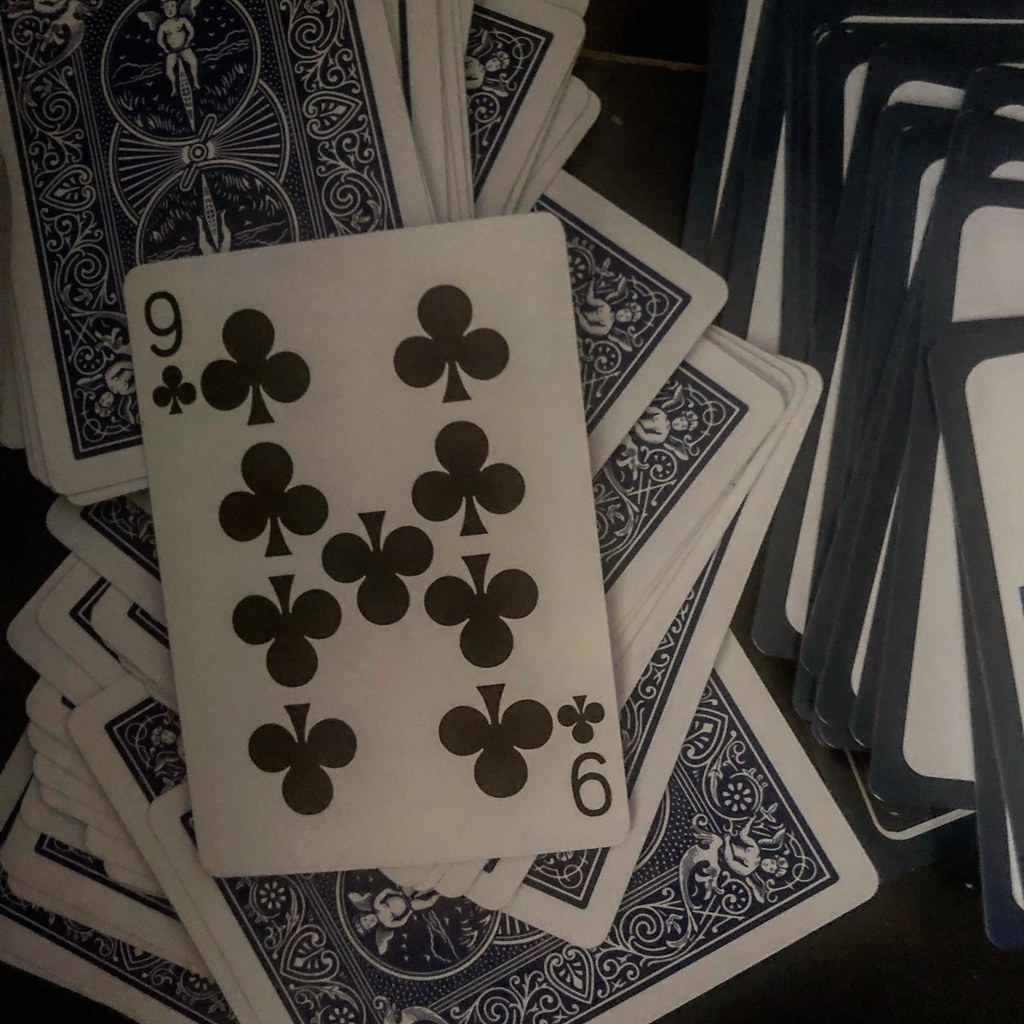This photo captures an intriguing collection of playing cards casually arranged in a seemingly haphazard pile. To the right, a pack of cards flaunts a vivacious design on its back, featuring a cyclist, abstract geometric shapes, and an elaborate mandala motif. The pack, marked by intricate and colorful artistry, prominently displays the Nine of Clubs on top. This card, rendered in classic design, showcases nine black clubs against a white background, with the number '9' positioned at the top left and bottom right corners. Adjacent to this striking pack lies another set of cards, partially visible and sporting a sleek black border against a white background. Though their details remain obscured, both packs rest on a dark tabletop, accentuating their vivid designs and chaotic arrangement.